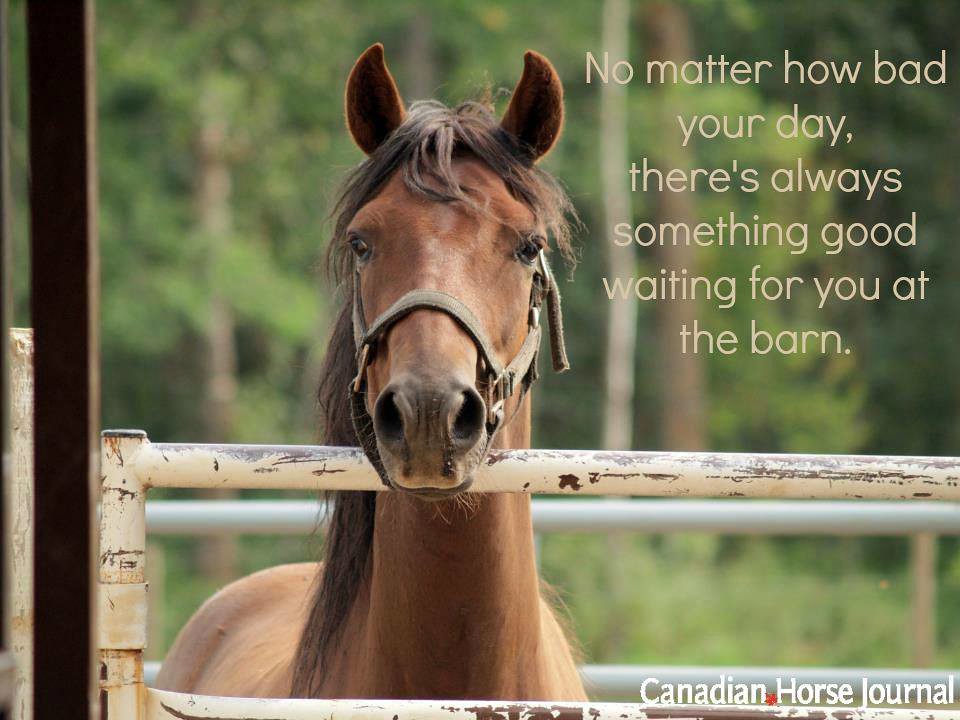In this captivating image, a brown horse with a bridle, but no bit in its mouth, stands prominently against a green background. The horse's head is raised and resting gently over a faded, chipped white metal fence that stretches horizontally across the picture. His attentive eyes gaze directly into the camera, capturing a moment of quiet anticipation. Behind the horse, there's a mixture of green grass and tall trees, including what appears to be a large trunk and possibly pines in the backdrop, contributing to a serene, natural setting. The top half of the horse is visible, displaying his neck, ears, mane, and part of his back, but his legs remain out of sight. In the upper right corner of the image, a comforting message in white font reads, "No matter how bad your day, there's always something good waiting for you at the barn," with a capital "N" and the rest in lowercase, ending with a period. Additionally, in the lower right corner, the text "Canadian Horse Journal" is neatly displayed, also in white font. Both elements of text harmonize with the tranquil and hopeful ambiance of the photo.